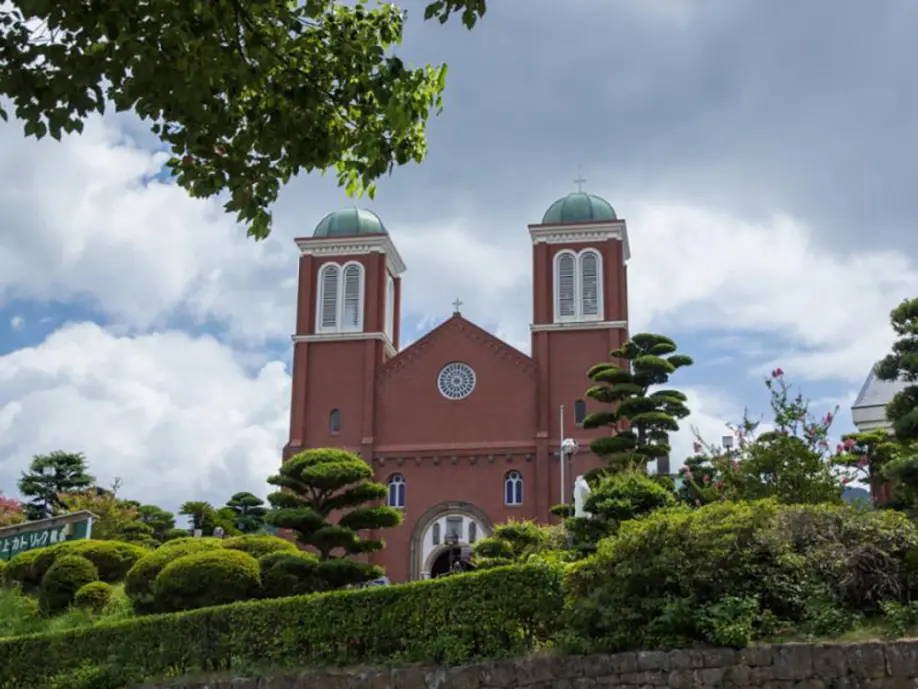The image captures a picturesque photograph of a reddish-brown church from a slightly lower perspective, situated along a street level with an elevated path leading towards it. The church boasts two prominent towers flanking the main entrance, each adorned with large white arched windows and capped with light blue dome roofs, each featuring a cross at the pinnacle. Central to the church’s façade is a majestic main arching door, above which another cross is positioned at the midpoint of the roof, adding to the ecclesiastical charm.

In the foreground, meticulously maintained plants, bushes, and small trees surround the church, indicating careful upkeep by a gardener. A stone fence and a well-groomed hedge border the area, suggesting a well-curated landscape. To the far left of the frame, a green sign with white Japanese symbols adds a unique cultural touch.

The backdrop features a partly cloudy sky with puffy, positive-looking clouds, casting a soft light over the scene, while tree branches in the upper left corner subtly intrude into the frame, enhancing the natural, serene ambiance of the photograph.